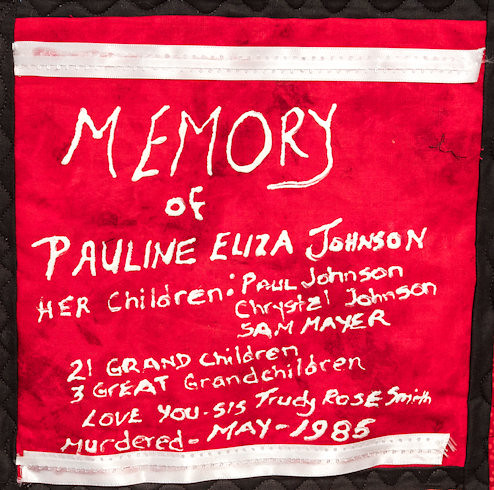This image depicts a poignant memorial banner with a handmade touch. Against a black patterned background, the magenta-reddish banner stands out prominently. A straight white border decorates the top, and a wavy white border graces the bottom. At the very top, in large white letters, the word "Memory" commands attention. Below it, centered, the banner reads "Memory of Pauline Eliza Johnson." 

The banner enumerates her loved ones explicitly: "Her children: Paul Johnson, Crystal Johnson, and Sam Mayer." Following this, it lists "21 grandchildren" and "3 great-grandchildren." A heartfelt message, "Love you," is also included, attributed to "Sis Trudy Rose Smith." The memorial concludes somberly with the distressing detail, "Murdered May 1985," accentuated by another white wavy banner at the bottom. The handcrafted tribute speaks volumes of the love and remembrance her family holds for her, despite the tragic circumstances of her passing.